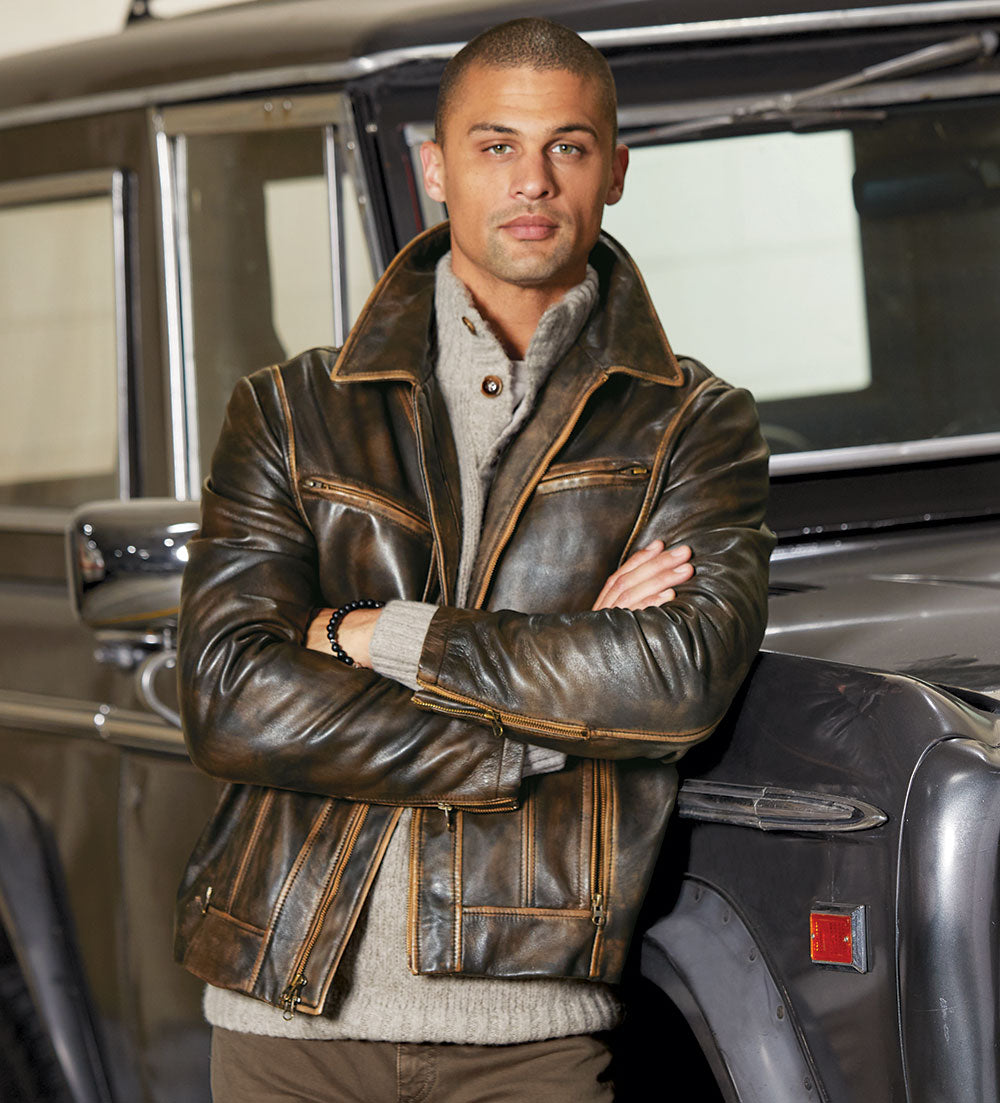The photograph captures a young Black man in his late 20s, standing outdoors, leaning against the back of a silver pickup truck. He has short, dark hair and light brown skin, with the beginnings of a mustache and beard. His arms are crossed, giving him a composed and confident look as he gazes directly at the camera, without a smile. He’s clad in a stylish brown leather jacket that has varied shades of brown, layered over a thick, gray button-down sweater. On his left wrist, he wears a set of black beads, reminiscent of prayer beads. The setting appears slightly vintage, evoking a sense of nostalgia with the old-style truck, which has a visible red reflector in the bottom right-hand corner of the frame. The cab of another truck can be seen in the top left-hand corner, grounding the scene in a practical, everyday environment. This image, richly detailed, frames the man almost as a stoic, modern-day hero, exuding strength and resilience.